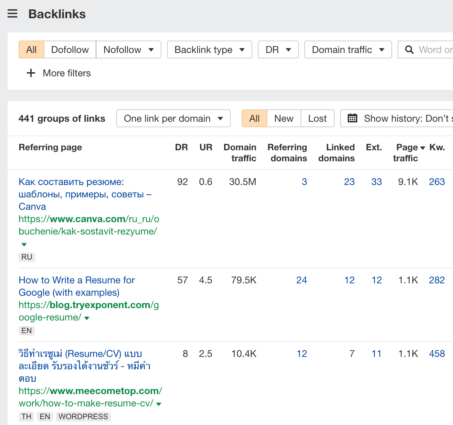This image displays a user interface centered on backlink analysis. At the top, the word "backlinks" is prominently featured in bold black font against a gray background. Below this, there are three straight lines, followed by filter options labeled "All," "Do Follow," "No Follow," "Link Type," "DR," "Domain Traffic," and a magnifying glass icon serving as a search function. Adjacent to these, there's a plus sign and the text "More Filters."

Further down, the image indicates "441 groups of links, one link per domain" with options "All New," "Lost," "Show History," and an accompanying calendar icon. 

Next, there are column headers: "Referring Page," "DR," "UR," "Domain Traffic," "Referring Domains," "Linked Domains," "External Page Traffic," and "KW." Among these, some entries are in the Russian language, while a link titled "How to Write a Resume for Google with Examples" appears in blue font. Additional text in Thai language is visible as well.

The interface primarily features a white background, with hyperlinks to websites displayed in green font. This concludes the detailed overview of the image.